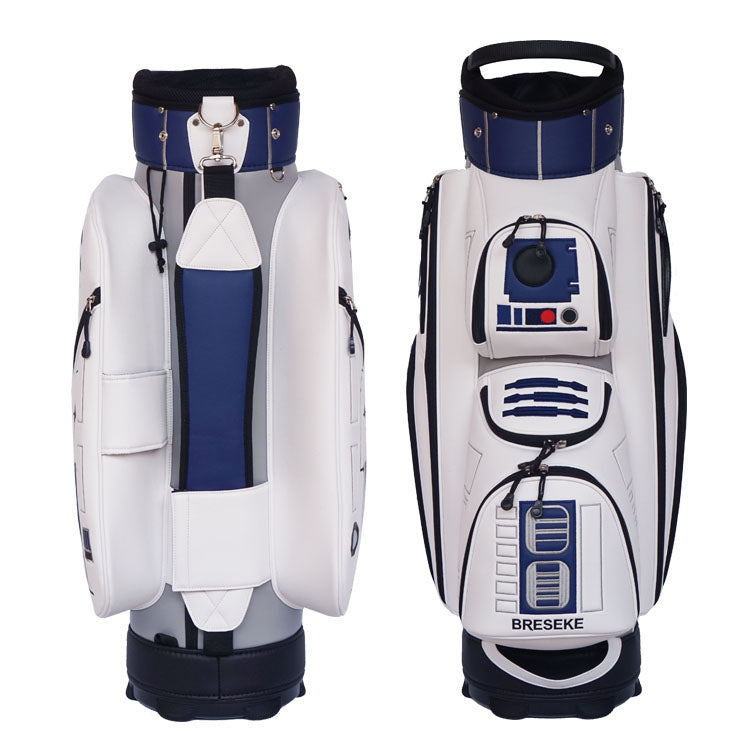The image displays a uniquely designed bag reminiscent of R2-D2 from Star Wars, featuring a front and back view. The bag has a predominantly white base with blue and black accents throughout and is laid out against a white background. The front displays a robotic design with a red button akin to an interface panel, a prominent black eye, and numerous dark blue details, lending it a strikingly futuristic look. Silver buckles and black zippers adorn various pockets, adding to the intricate detailing. The brand name "Bresci" is visible on the back, and "B-R-E-S-E-K-E" is noted on a compartment towards the bottom. The bag includes blue straps and a handle on top, further enhancing its utility.